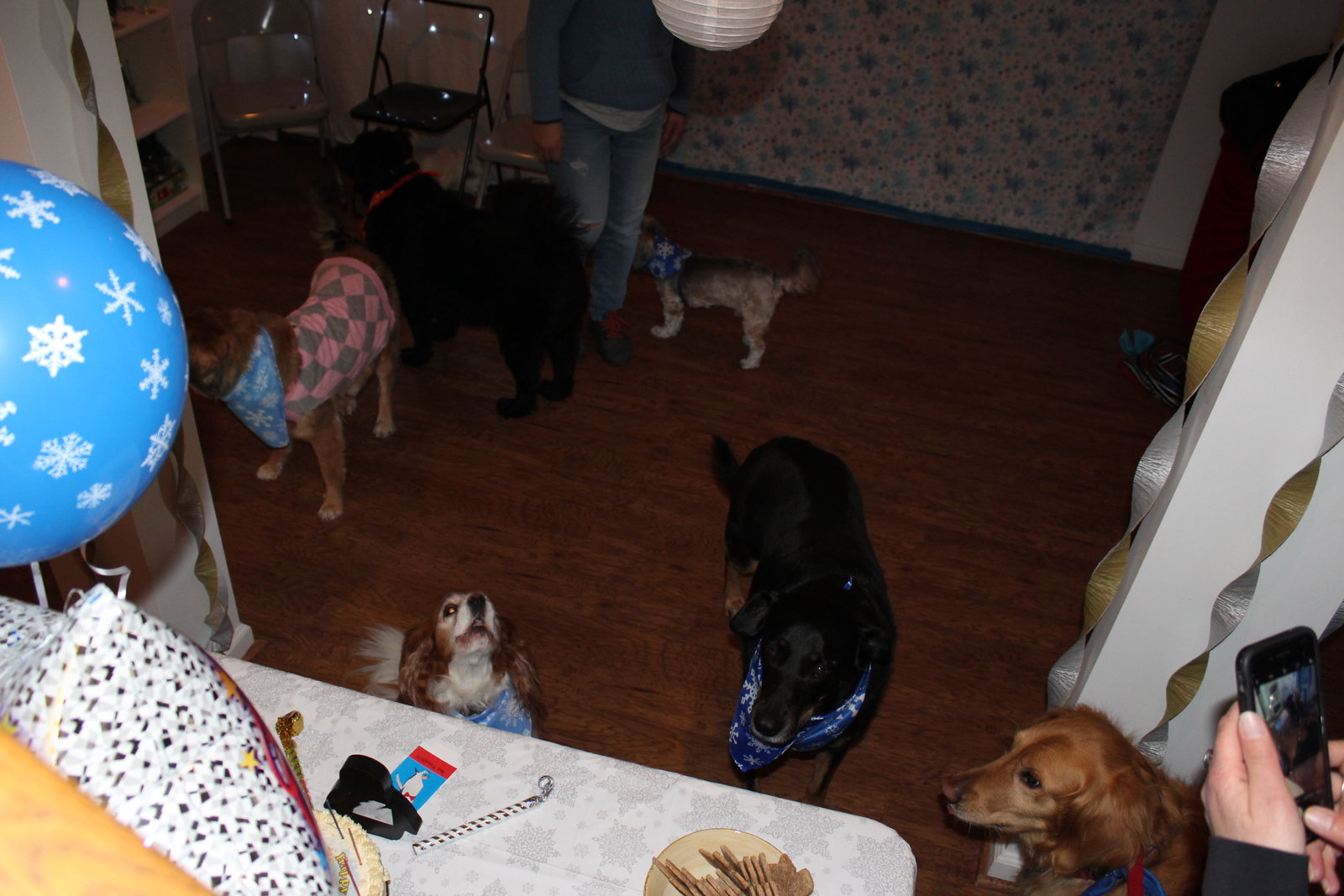The photograph depicts a whimsical dog birthday party set in a dimly lit living area with a touch of holiday spirit. The wooden floor is adorned with several dogs of various breeds, each sporting bandanas featuring snowflake patterns. Among the dogs are a golden retriever, a black shepherd, a terrier, and a fluffy black dog, all wearing their festive accessories. 

On the left side, a table dressed with a white tablecloth also embellished with snowflakes holds several party essentials including a dish of dog treats and a birthday cake partially hidden from view. A large blue balloon with white snowflakes complements the theme and ties in with the blue bandanas worn by the dogs. 

In the background, a person in blue pants and a matching hoodie stands by three folding chairs—two gray and one black—while another person in the bottom right corner, with only their hands visible, captures the moment on their phone. The wall features a gray patterned wallpaper with blue details, adding to the cozy atmosphere. Silver and gold streamers dangle from the ceiling, enhancing the festive environment.